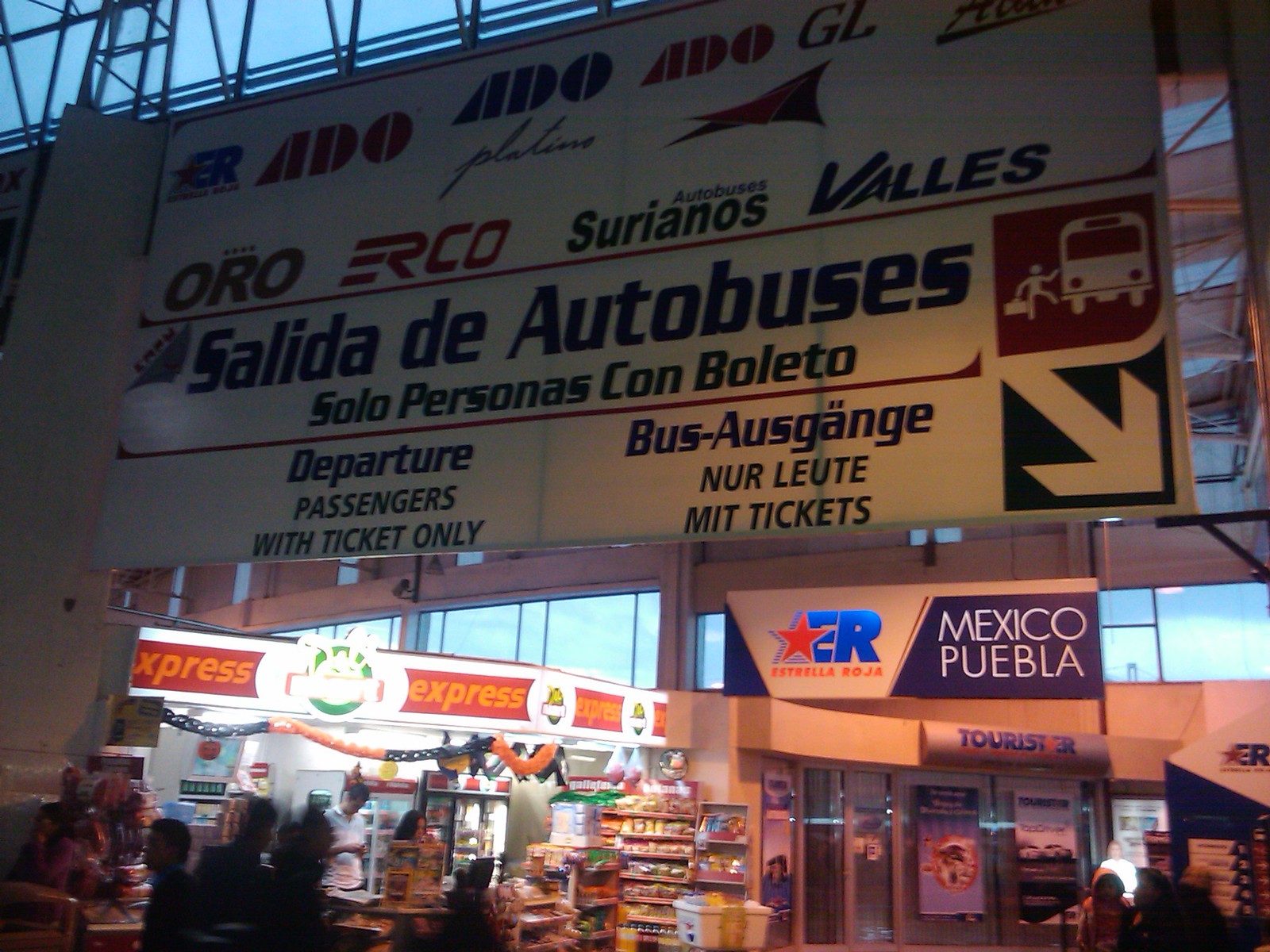The photo depicts the entrance of a transportation center, likely a major bus station in Mexico. Dominating the scene is a large white sign that reads "Salida de autobuses, solo personas con boleto," accompanied by an icon of a person boarding or alighting a bus, carrying a suitcase, with an arrow pointing down to the right. Below this, the sign indicates the destination: "Mexico Puebla". To the left of the sign, there's a star emblem with the letters "ER" and the name "Estrella Roja."

In the bottom left corner of the photo, a convenience store or food station is visible, brightly lit with red and green neon lights, offering food for purchase. The station's high ceilings and numerous windows suggest a spacious, airport-like atmosphere, though the lighting appears somewhat dim. The setting is bustling and geared towards travelers, emphasizing the organized structure of the transport hub.